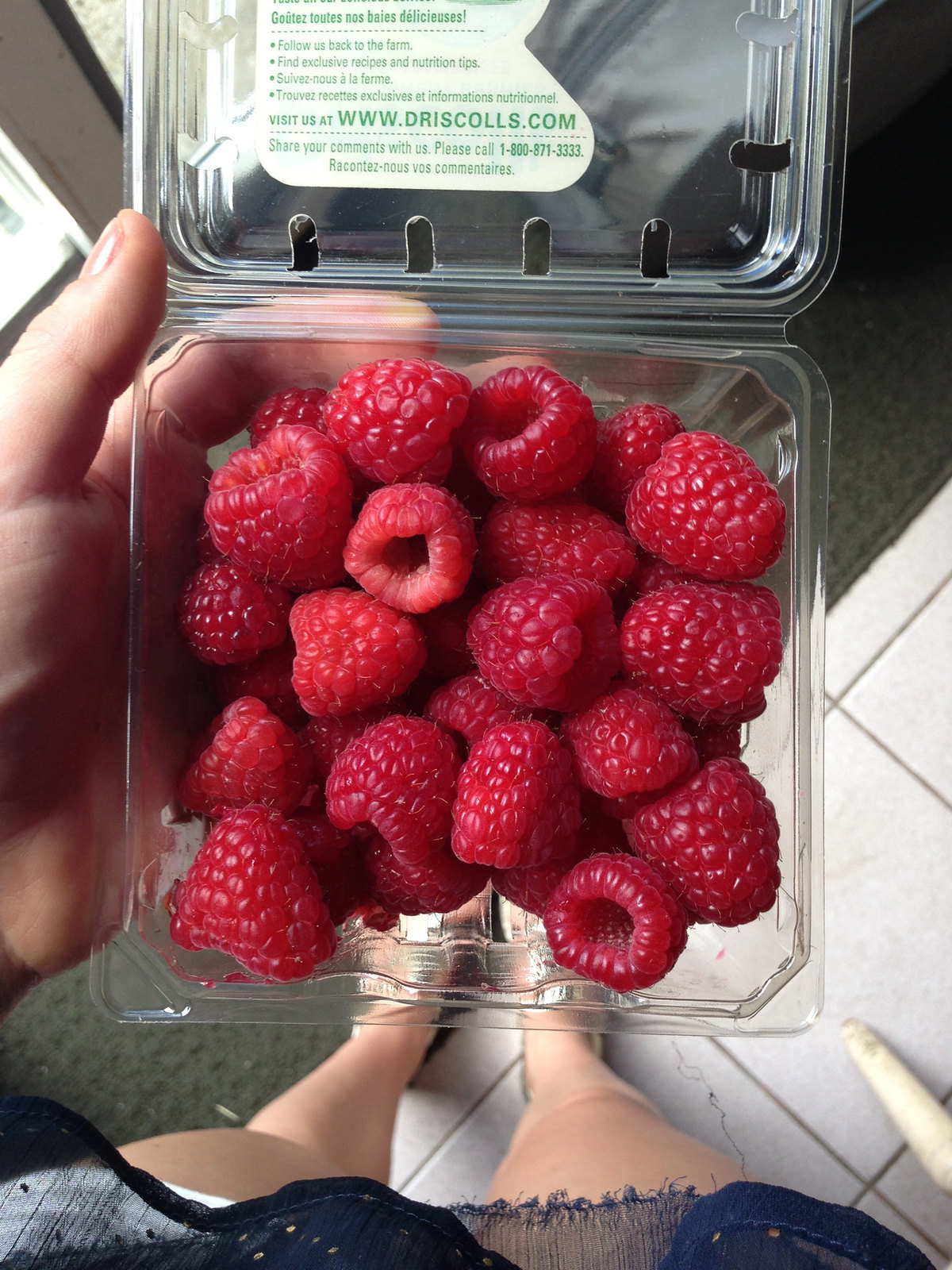This photograph features an overhead perspective of a woman holding a clear plastic container of fresh, bright red Driscoll's raspberries. The container, which appears to be half a pint, prominently displays a label in both English and French encouraging consumers to visit www.driscolls.com for exclusive recipes and nutrition tips, and to call 1-800-871-3333 for comments. The woman, identifiable by her bare legs and white sandals, is clad in a blue gauzy, lacy shirt with white shorts underneath. She holds the raspberries in her left hand while standing on a white tiled floor next to a metal grate, possibly outside in front of a store. The scene also includes the edge of a dark green or olive-colored rug.